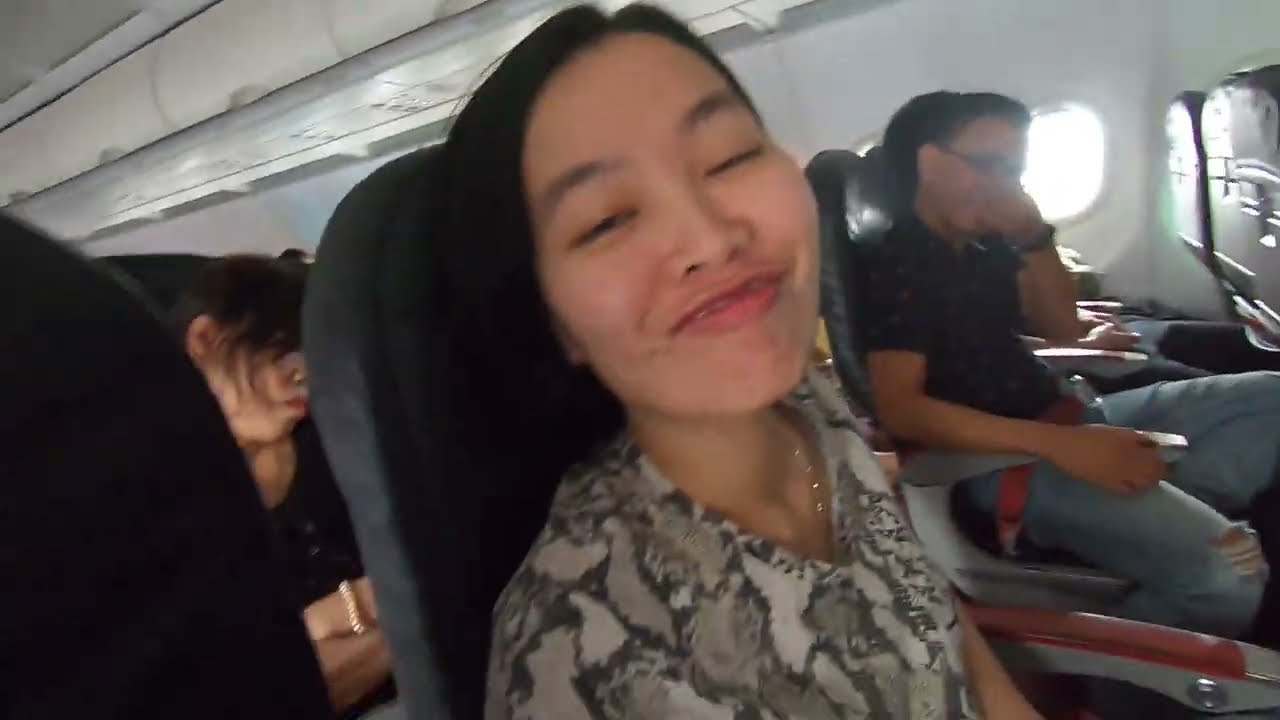This horizontally aligned rectangular image, though slightly blurry, captures a close-up of a young Asian woman inside an airplane. She has long, straight black hair and is wearing a patterned gray and white blouse reminiscent of snakeskin, partially revealing a necklace chain. Her expression is playful, characterized by a goofy smile with her mouth slightly open and her eyes squinted, almost closed, as she looks directly at the camera, suggesting that she is taking a selfie. 

Behind her, another woman, possibly asleep with her head bowed, is visible wearing a black top and a bracelet, and has her arms folded. To the right of her in the photo, there's a man sitting by the airplane window. He is dressed in a short-sleeved black patterned shirt and light blue jeans, torn at the knee, with a red seat belt across his waist. The background showcases the airplane's white ceiling and walls, overhead luggage compartments, and black seats. The bright light from the windows hints that it is daytime outside.